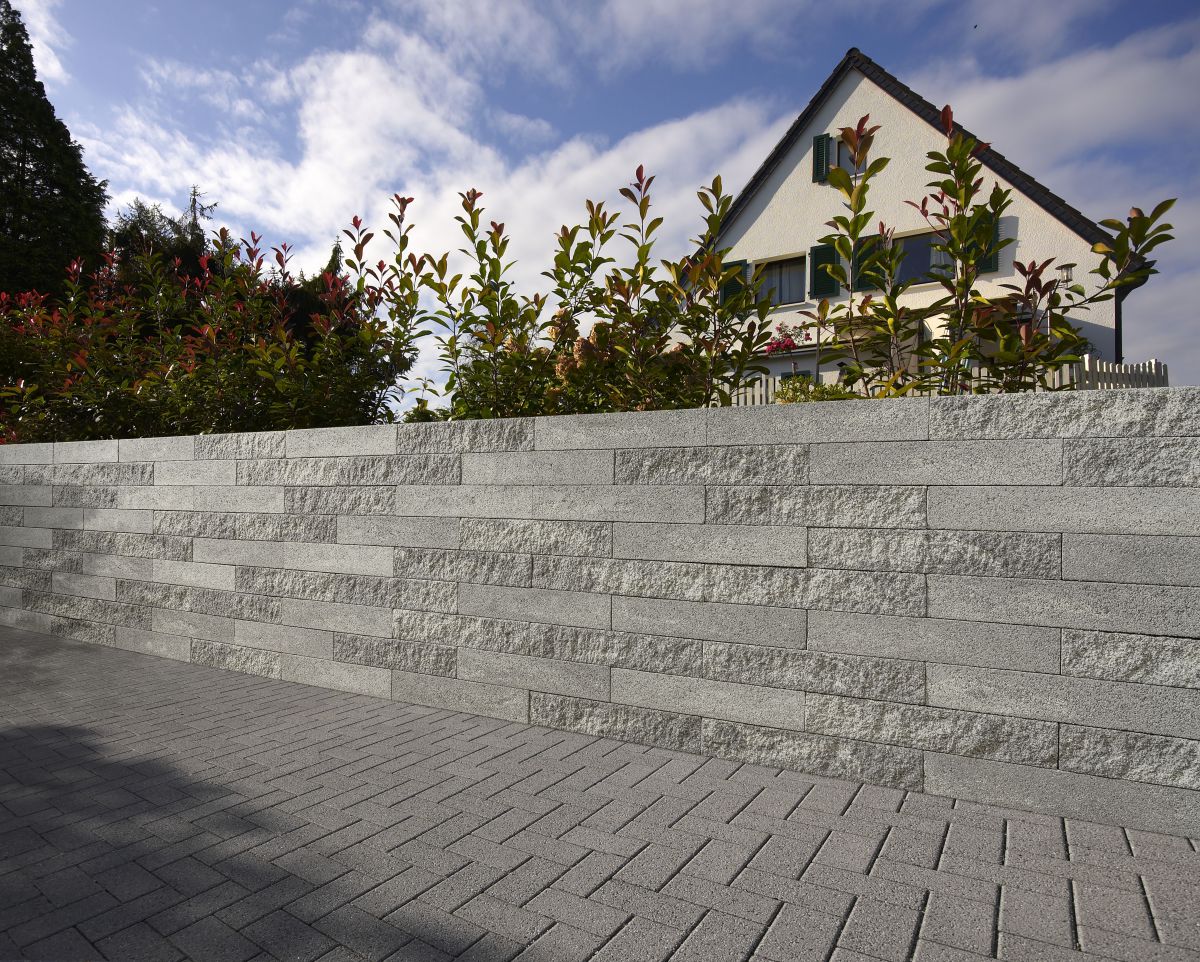The image depicts the front of a residential house partially obscured by an abundance of foliage. In the foreground, there is a gray brick sidewalk leading up to a substantial wall, possibly made of concrete or brick, that appears to serve as a fence. The house itself has a cream-colored exterior with a dark roof and three windows on its upper level. To the right side of the image, the house is more visible, partially hidden behind tall trees and dense shrubbery, allowing just glimpses of the windows and walls. On the left side, additional trees add to the lush surroundings. The background reveals a bright, cloudy blue sky. Dominant colors in the scene include green from the foliage, blue from the sky, and muted tones of white, gray, and brown from the architecture and natural elements.